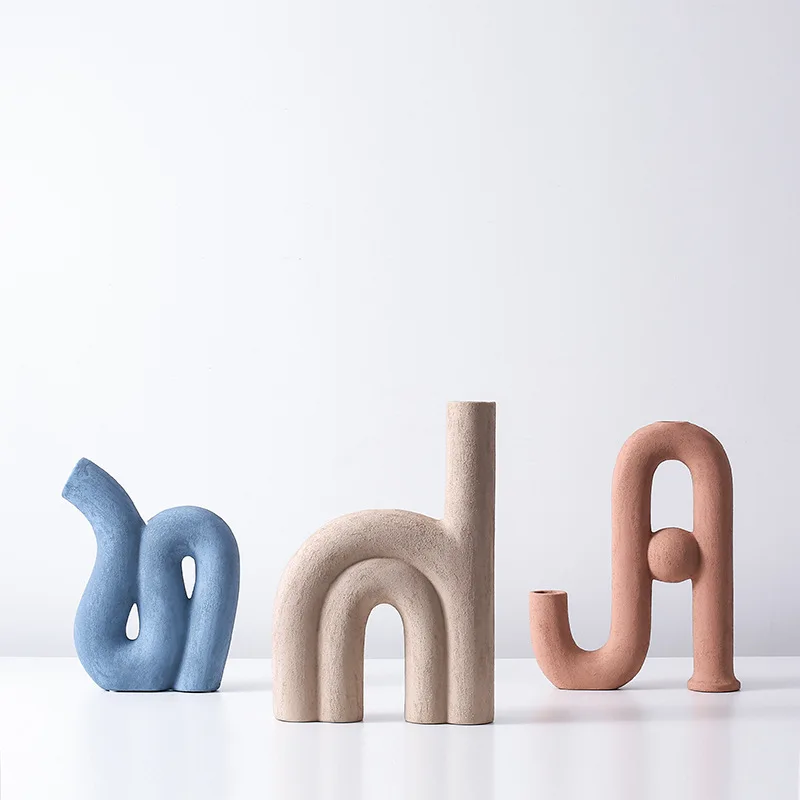The image showcases a professionally taken photograph of three abstract clay sculptures arranged on a reflective white surface set against a slightly grayish background that fades to white in the lower left corner. The sculptures are hollow and tube-like in form, each exhibiting unique shapes and colors. 

On the left, the sculpture is light blue and resembles a coiled line, curving down, up, and down like a stylized, abstract representation of a snake or an inverted U with an elongated snout. In the center, the sculpture is light pink (some describe it as light brown or white) and resembles a backwards H with a secondary level shaped like an N beneath it. On the right, the sculpture is a darker pink or orange, and resembles a twisted water pipe or a J, featuring a bowl-like form in the middle of its curve.

The lighting is excellent, highlighting the shadows and reflections on the white surface, enhancing the intricate details of each piece. The image captures the essence of abstract art, inviting multiple interpretations of these hollow, tube-like clay sculptures.